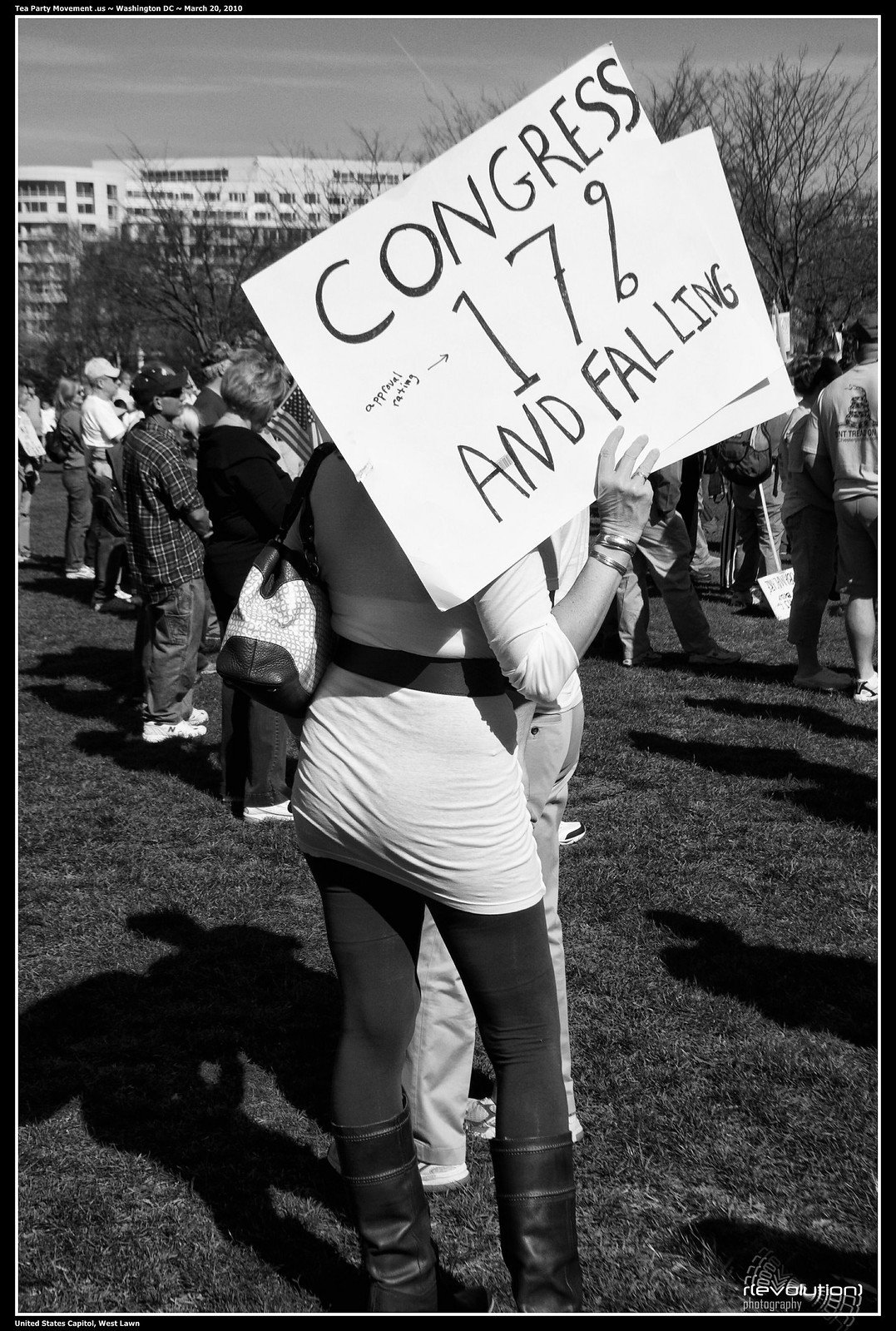In this detailed black-and-white photograph set within a distinct black border, the scene unfolds on the West Lawn of the United States Capitol, as indicated by the watermark reading "Tea Party Movement, Washington, D.C., March 20th, 2010." The image captures a vintage moment at what appears to be a protest or rally. In the center foreground, a woman dressed in a white top and short white skirt, complemented by black leggings and boots, stands with her back turned to the viewer, holding a large white sign emblazoned with the bold black text, "Congress, 17% and falling." An arrow points to the "17%" with the notation "approval rating," emphasizing the message she wishes to convey. A purse hangs over her left shoulder, adding to her distinct silhouette. 

The event takes place on a grass field, with the soft shadows of various participants falling onto the ground. Scattered around are people, some holding signs mounted on wooden sticks, hinting at the collective sentiments of the assembly. In the middle ground, one individual prominently waves an American flag. The crisp outlines of several barren trees stand out against the sky, devoid of leaves, adding to the starkness of the scene. The large white Capitol building looms in the background, giving context to the protest's location, its multiple stories clearly visible. The photograph itself is credited to "Revolution Photography," as seen in the bottom right watermark. The striking details of the image capture a momentous gathering, highlighting public dissent towards the U.S. Congress's low approval rating at that time.